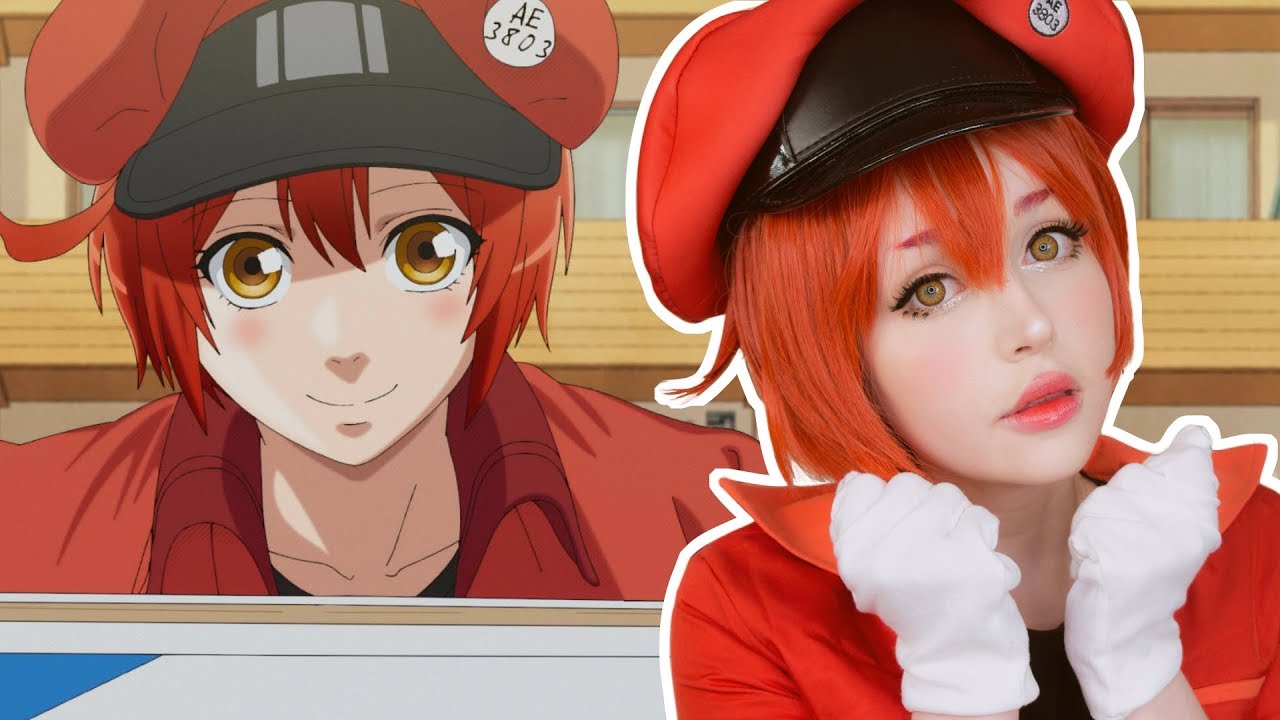This image features a side-by-side comparison of a cosplayer and the anime character she is portraying. On the left-hand side, the anime character is depicted with vibrant red, short hair, large amber eyes, and a red hat adorned with the identifier "AE-3803." She wears a red coat, a black top, and white gloves. The cosplayer on the right mirrors this look precisely. She is a Caucasian woman with short, striking red hair, either dyed or a wig, and wears amber contact lenses to match the character's eye color. Her cosplay includes the identical red hat marked with "AE-3803," a red coat, a black top, and white gloves. Additionally, there is a glimpse of a blue element in the corner of the image. Both the character and cosplayer exhibit meticulous attention to detail, making the resemblance striking and accurate.